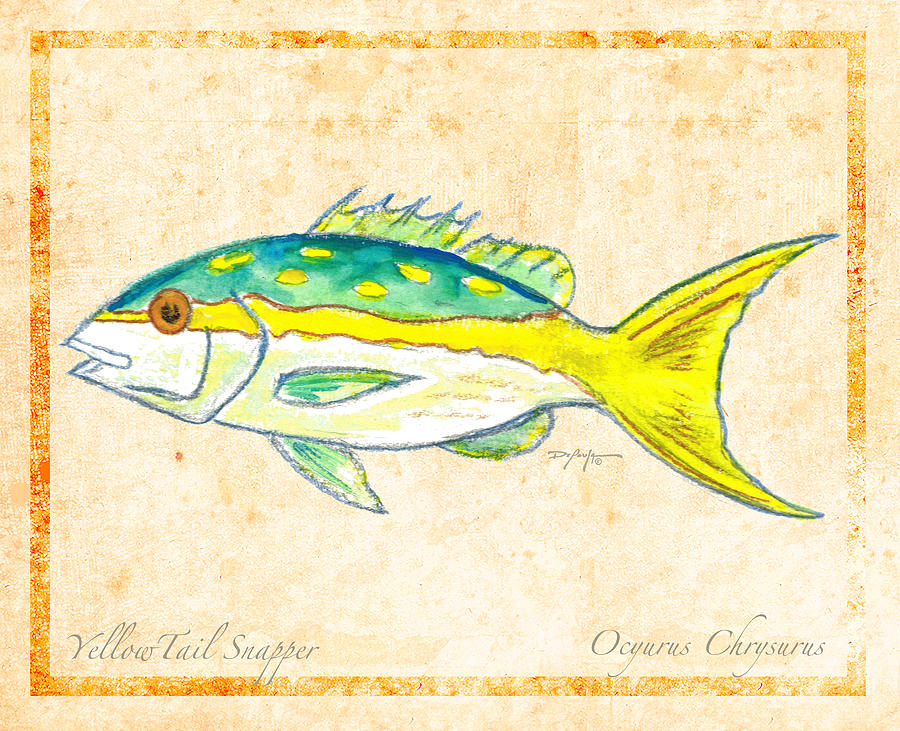This artwork displays a detailed illustration of a Yellowtail Snapper, depicted on a square canvas with a tan, papyrus-like background. The image features a vibrant fish with a dazzling array of colors, primarily green, yellow, teal, blue, and orange. Its tail is a striking green-yellow hue with red highlights, and its lower fins are a mix of green and white. The fish's top shows an aqua blue-to-green gradient adorned with yellow spots, and it includes a prominent dark orange or red eye.

The fish's name, "Yellowtail Snapper," is elegantly written in cursive in the bottom left-hand corner, while "Acurus Chrysorus" (or similar variations) appears in the bottom right. This inkling aligns with the highly detailed border surrounding the fish; a rich orange or red line encapsulates the drawing, enhancing the crayon or pastel-like shading and giving it a well-composed and textured look. Near the tail, a small signature—presumably the artist’s—is subtly placed, adding a personal touch to the piece. The overall effect is a vibrant yet refined portrayal, likely completed with a combination of crayons or colored pencils that showcase depth and meticulous attention to detail.